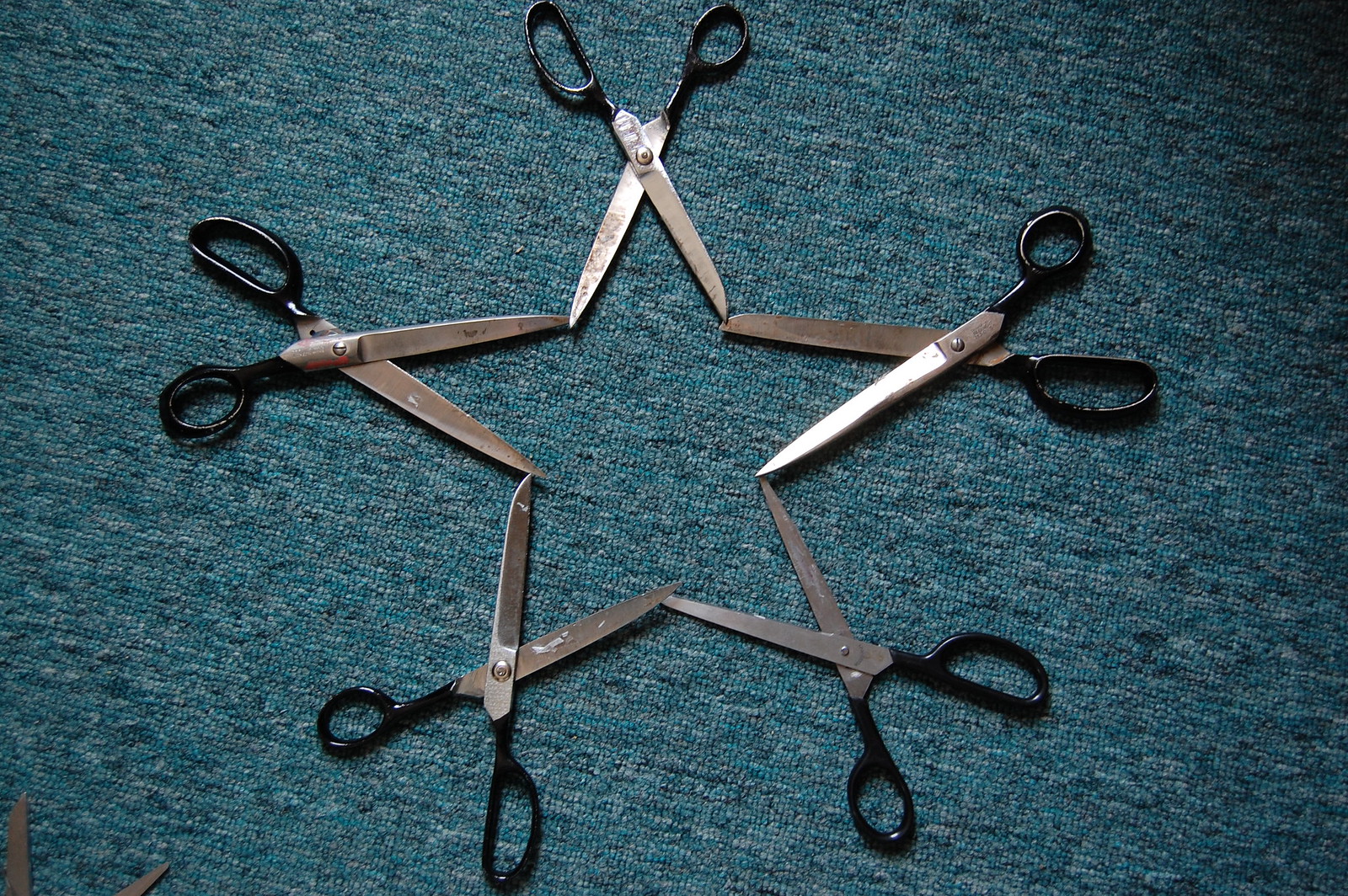The photograph captures a top-down view of a teal blue carpet with flecks of black and white, possibly an indoor-outdoor-style rug. Arranged meticulously on the carpet are five pairs of black-handled, silver-bladed scissors, slightly open to form a five-pointed star. The blades of the scissors, though largely reflective, feature some spots of white residue and signs of rust, giving them a somewhat aged appearance. The handles are black and extend halfway down the blades, which are held together by round screws. At the bottom left corner, the tip of another pair of scissors is just visible, hinting at a larger collection. The composition is reminiscent of a Busby Berkeley geometric arrangement, lending a touch of artistry to the everyday objects.